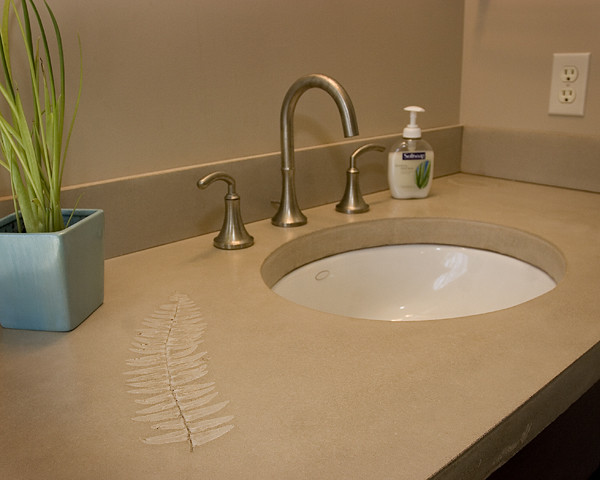The photograph features a bathroom sink area captured from a slightly left-angled perspective within a frame that is somewhat wider than it is tall. The sink, embedded in a brown countertop with an embedded leaf design on the left, extends diagonally across the image from the lower left corner toward about two-thirds up on the right-hand side. A curved faucet with two handles is centrally located above the white, recessed circular basin.

To the right of the faucet sits a container of Softsoap, while an electrical outlet is visible on the wall further to the right of the sink. On the left side of the vanity, a light blue, rectangular planter holds tall, green fronds, adding a touch of natural decor to the scene. The overall composition of the photograph thoughtfully captures these details, clearly indicating this is a bathroom sink area.